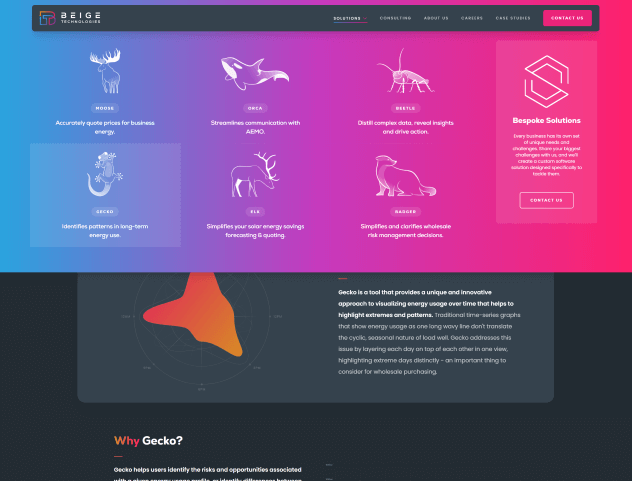This screenshot captures the homepage of AEIGE Technologies’ website. The website’s logo is prominently displayed in the upper left-hand corner. On the right side, there's a vertical menu that stands out with a vibrant color gradient transitioning from red to blue to purple. Adjacent to the menu, a series of images are aligned in a grid format.

The topmost row features three distinct images: starting with a picture of a moose, followed by an image of a whale, and concluding with a photograph of an insect. The subsequent row showcases a sequence of animal pictures, beginning with a salamander, followed by a deer, and ending with a fox.

Below these rows, the background subtly shifts to a gray hue. Positioned beneath this section, there's a light gray box containing an orange, circular blob that has a slightly muted, dull gray interior. The overall layout and color scheme create a dynamic and visually engaging interface.